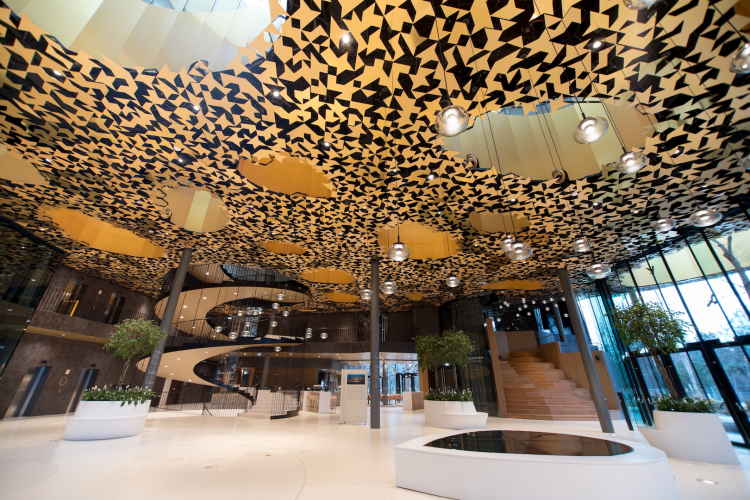The photograph captures an expansive, modern lobby bathed in an unusual yet playful ambiance. Distinguished by its rectangular shape, the image forefronts a polished, white-tiled floor adorned with multiple triangular seating areas hosting large white plants. On the lower right, the entrance features a series of pristine glass doors framed in black, beneath large glass panels that allow natural light to flood in.

Against the right wall, a brown stairway ascends to a mezzanine with a sleek railing, creating an inviting path to the upper level. To the left, a striking beige spiral staircase snakes elegantly upwards, connecting the ground floor to another level above in a visually compelling manner.

The ceiling is a testament to intricate design, adorned with geometric patterns of gold interspersed with black, resembling abstract star shapes. Despite its relatively low height, the ceiling features multiple openings that not only enhance the sense of vertical space but also allow glimpses into the upper level. Hanging lights descended from strings add a warmth and charm to the space, accentuating the ornate and patterned gold and black ceiling. This sophisticated design contrasts starkly yet harmoniously with the otherwise muted floor and wall tones, creating a dynamic and visually engaging lobby.